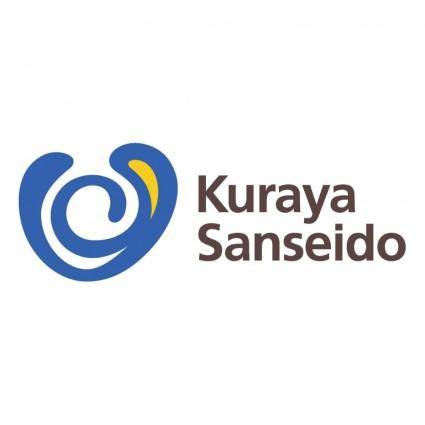On a solid white background with indistinct edges, there lies a central graphic that combines text and a logo. To the right, in a prominent dark brown font that almost appears black, are the words "Kuraya" on one line and "Sanseido" just below it. These words, possibly names, are written in capital K and S respectively, followed by lowercase letters. Taking up about 50% more height than the text to the right is a distinctive logo positioned slightly off-center to the left. The logo itself is a medium blue graphical element resembling an abstract U. Its shape is evocative of raindrops merging together, with a curve that begins at the top like an open V, bends down to form a partial at-sign, and where these curves converge, a yellow area is visible in the top right corner. This composition suggests the elegance and professionalism of a company emblem, potentially suited for use on business cards or company websites.